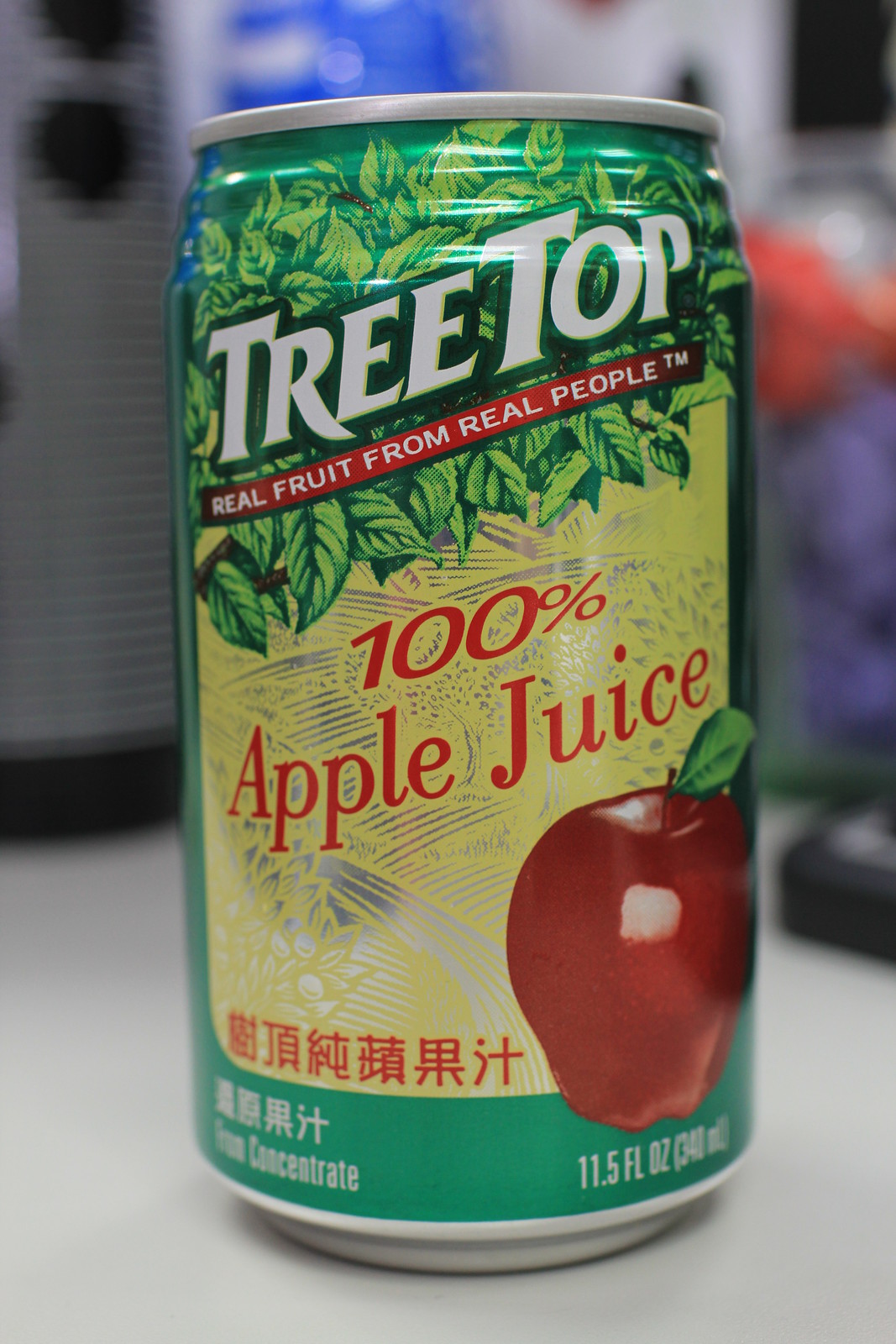This extreme close-up photograph captures a can of Treetop apple juice, a well-known brand. The image is taken indoors with a blurred background suggesting a dark room, with hints of white and black shapes. The can is metallic with a green-bordered label. At the top, the label features green leaves from a treetop. Bold white text reads "Treetop," followed by a red banner proclaiming "Real fruit from real people." The central part of the label, against a yellow backdrop depicting a farm scene with apple trees and hills, has red text stating "100% apple juice." An illustration of a large red apple is shown beneath, alongside some Asian Mandarin characters, indicating this product is targeted for the Asian market. Additional details include "from concentrate" and "11.5 fl oz" in smaller print. The can rests on a white table surface under bright indoor lighting.